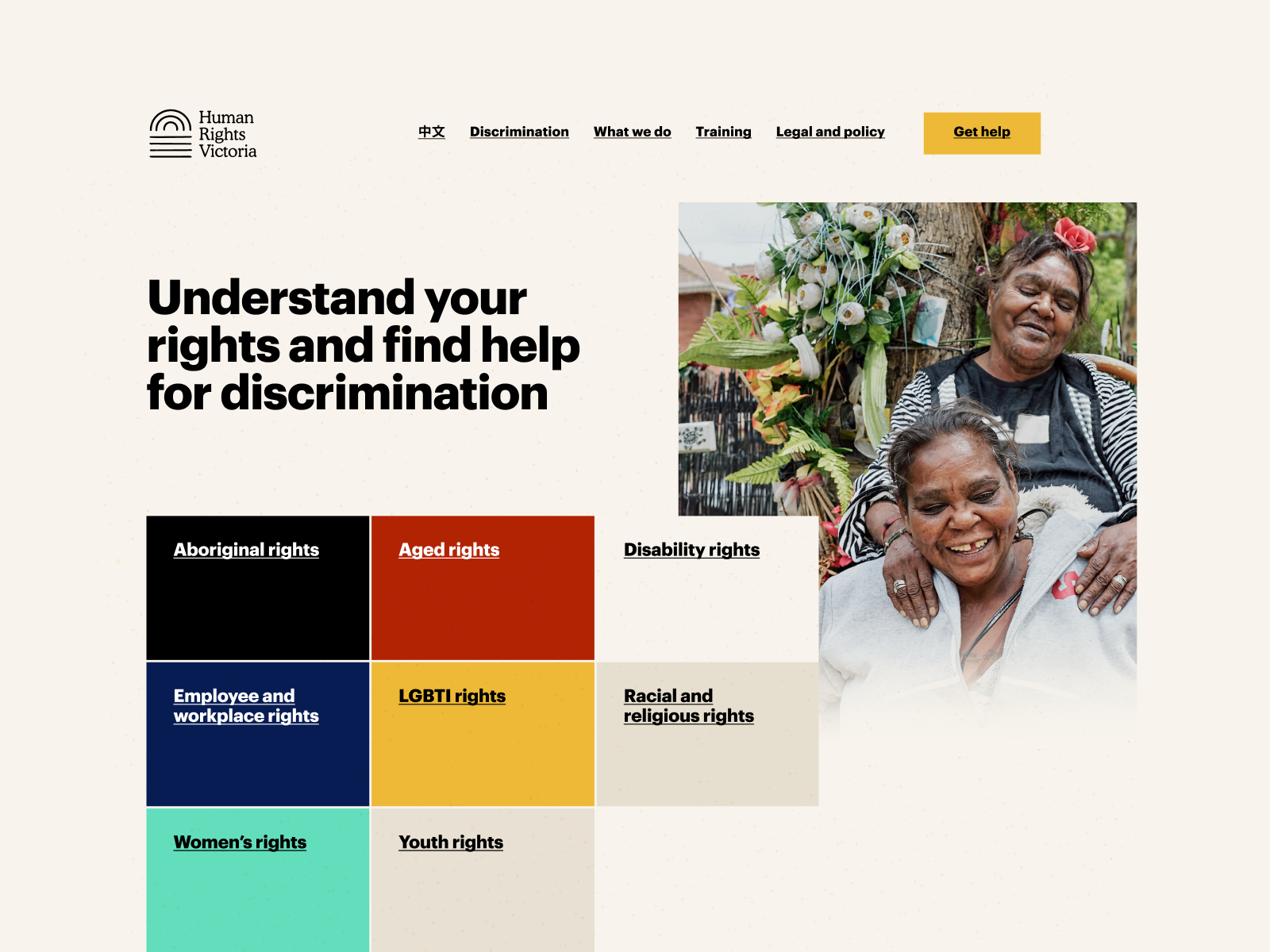In this detailed image of the Human Rights Victoria website, the logo is located in the upper left corner, featuring a half-circle dome design composed of three progressively smaller arcs stacked together. Below the logo, the text "Human Rights Victoria" is displayed with each initial letter (H, R, and V) capitalized.

The website's navigation categories include a language selection option, which appears to offer a Chinese translation. The main categories listed are: Discrimination, What We Do, Training, Legal and Policy, and a prominently highlighted "Get Help" category, which is underlined for emphasis. Just below the logo, in bold black letters, the text reads: "Understand your rights and find help for discrimination."

To the right of the logo, there is an image depicting two women, one standing and one sitting, who appear to be of Aboriginal heritage. Adjacent to this image are eight distinct colored boxes, each representing a different category: 
1. Aboriginal Rights (black)
2. Aged Rights (red)
3. Disability Rights (white)
4. Employee and Workplace Rights (blue)
5. LGBTI Rights (yellow)
6. Racial and Religious Rights (gray)
7. Women's Rights (green)
8. Youth Rights (gray)

These boxes serve as clickable links that direct users to more specific information within each rights category.